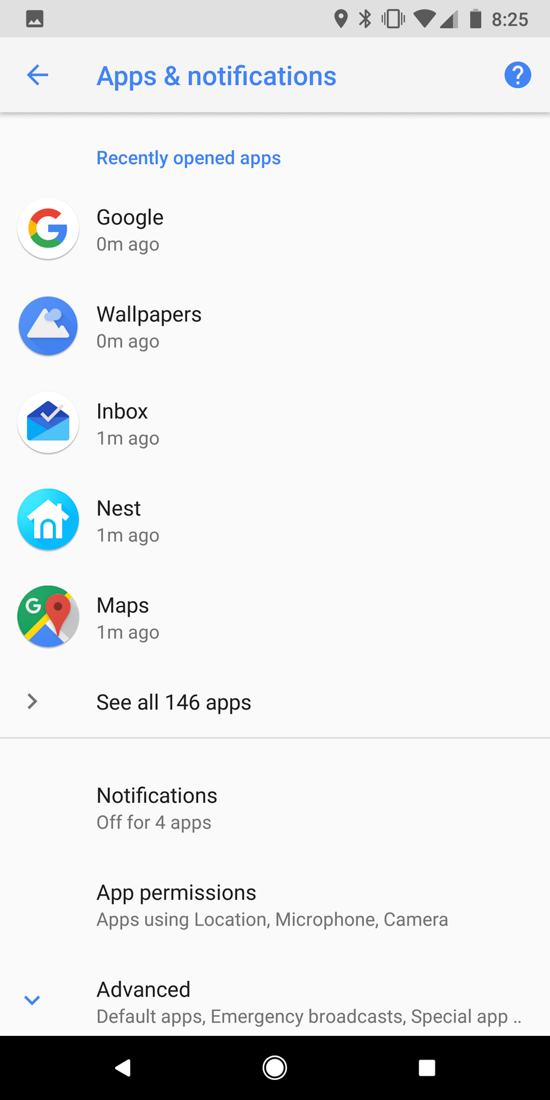The image depicts a smartphone screen displaying the "Apps & Notifications" settings menu. 

At the top left corner is an ambiguous black and gray icon, possibly resembling a map. The status bar at the top of the screen shows various black icons including location services, Bluetooth, Wi-Fi, signal strength, and battery life indicators, alongside the current time "8:25," all set on a light gray background.

The page header, "Apps & Notifications," appears in blue text at the top, accompanied by a blue circle with a white question mark within it, suggesting access to additional information. To the left of the header is a blue left arrow, indicating a navigation option to return to the previous screen.

Just below the header, a smaller blue text reads "Recently opened apps," followed by a list of apps with respective icons and the times they were last opened:
1. **Google**: Recently opened, with its iconic multi-color 'G' logo.
2. **Wallpapers**: Also recently opened, represented by an icon featuring a mountain and a moon or sun against a blue background.
3. **Inbox**: Opened one minute ago, marked by a blue envelope with a checkmark on a white circle background.
4. **Nest**: Opened one minute ago, denoted by a white house icon set against a light blue circle.
5. **Maps**: Opened one minute ago, featuring the classic Google Maps pin icon.

Below this list, the text "See all 146 apps" appears with a right arrow, implying further navigation to view all installed apps. A thin horizontal gray line separates this section from additional menu options.

Further down, the screen indicates various settings and statuses:
- Notifications turned off for four apps
- App permissions, detailing apps using location, microphone, and camera
- An advanced settings section with options such as default apps, emergency broadcasts, and special app access, indicated by a downward arrow suggesting it is already expanded.

The image truncates at the bottom, where a black navigation bar displays a back arrow, a home button, and an overview button, rounding out the standard smartphone interface.